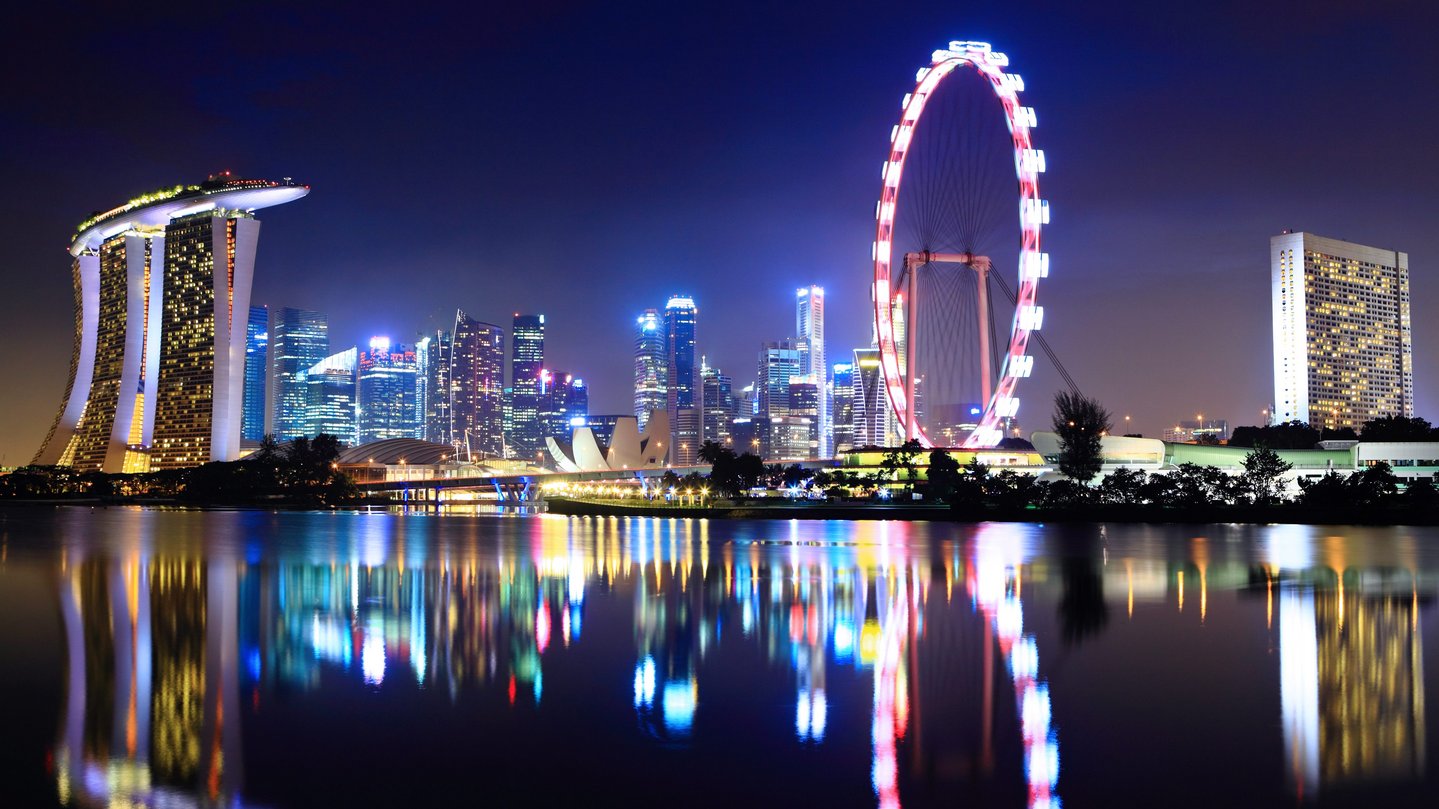This is a breathtaking nighttime cityscape featuring a vibrant, futuristic metropolis viewed from across a body of water, likely a river or large lake. In the center of the image stands a giant, brightly lit Ferris wheel, its red and blue lights casting vivid reflections onto the water below. To the left, a striking building with three distinct supports and a UFO-like appearance dominates the view, its numerous lights illuminating the scene. The city backdrop is composed of a myriad of uniquely shaped skyscrapers, their multicolored lights—including hues of blue, red, yellow, and orange—creating a stunning rainbow-like effect across the skyline. On the far right, a high-rise building, possibly a hotel or casino, is visible. This building's partial illumination suggests it might be occupied by offices or apartments. Additionally, a statue resembling an opening flower is located on the opposite side of the water. The collective effect of these dazzling lights reflecting on the serene water surface creates a beautiful, almost double image, contributing to the city's modern and forward-looking ambiance.